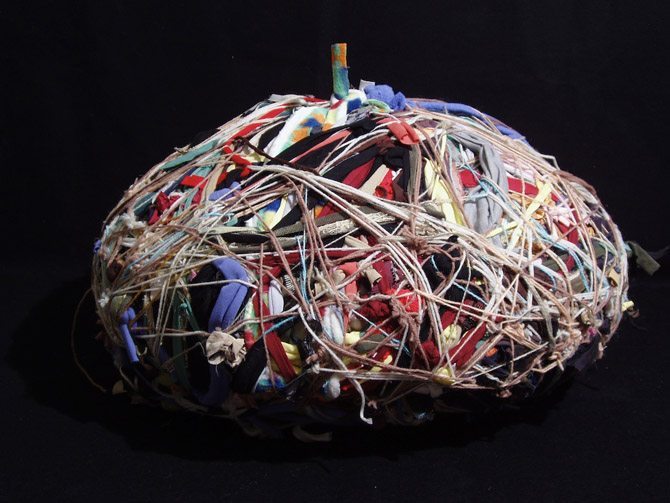In this detailed multimedia art piece, a massive, spherical ball of twine, yarn, string, and various fabrics, including articles of clothing, is showcased. The ball features an eclectic mix of colors—red, blue, beige, white, coral, gray, tan, orange, yellow, green, purple, pink, black—with thicker ribbons of blue and thin strands of red standing out. Predominantly beige and white burlap-style twine interlaces among these vibrant materials. At the very top of the ball, a thin one-inch wooden peg, painted green, protrudes. The sculpture is set against a shiny, pitch-black backdrop and rests on a black table, accentuating the ball's chaotic yet captivating design. The entire composition is centered within a nearly square, horizontally rectangular frame, emphasizing the unpatterned, haphazard manner in which the materials are intertwined, giving the piece a visually dynamic and richly textured appearance.